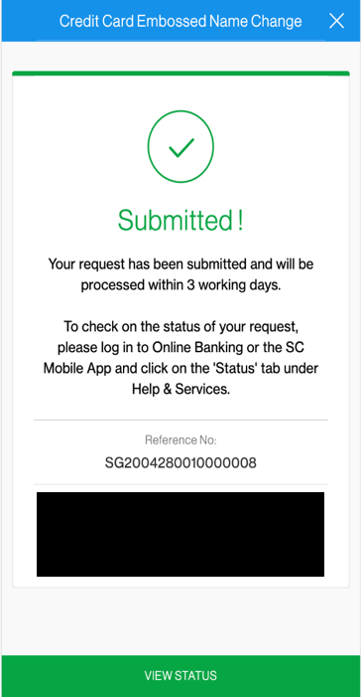This image is a screenshot from a mobile banking app on a cell phone. The user interface predominantly features a white background. At the top, a light blue banner spans the width of the screen, displaying the text "Credit Card Embossed Name Change" in white, accompanied by a white "X" icon on the right for closing the page.

Below this banner, there is a thin green line followed by a green circle set against a white background, containing a white check mark in the center. Beneath this icon, the text "Submitted!" is prominently displayed in green.

Further down, in smaller black text, the message reads: "Your request has been submitted and will be processed within three working days. To check on the status of your request, please log into online banking or the SC Mobile app and click on the Status tab under Help and Services."

A long alphanumeric reference number is shown below this message, partially obscured by a large black rectangle, likely added to conceal personal information.

At the very bottom of the screen, a green bar with the text "View Status" in white invites users to check the status of their request.